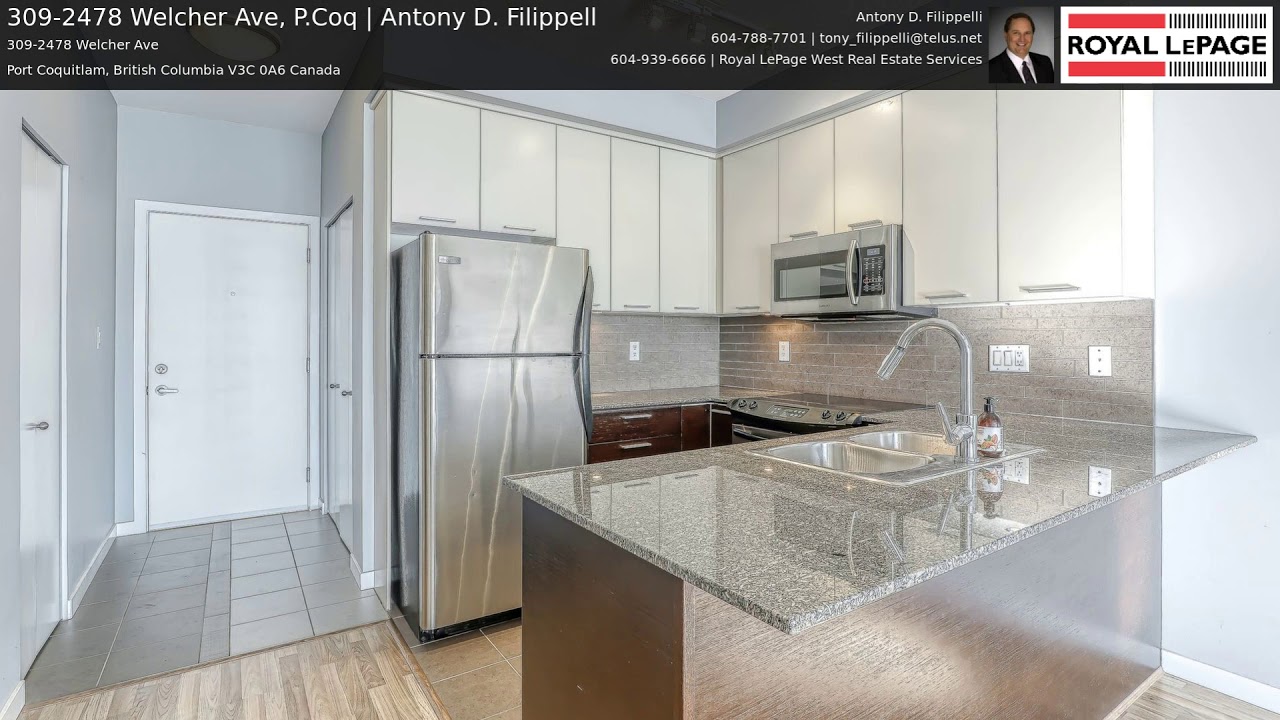A screenshot of a real estate advertisement page features a modern kitchen at the bottom. The kitchen includes a gray granite countertop, a silver refrigerator with the freezer on top, and white cabinets. To the left, there is an entryway with gray tile flooring leading into the kitchen area, which has brown tile flooring. A section of wood flooring is visible in the bottom left corner of the image. The top of the page has a black horizontal banner with the text: "309-2478 Welcher Avenue, P.COQ, Anthony D. Philippal, 309-2478 Welcher Avenue, Port Coquitlam, British Columbia, V3C 0A6, Canada." On the right side of the banner is a photograph of Anthony D. Philippal. The Royal LePage logo is positioned in the upper right corner.